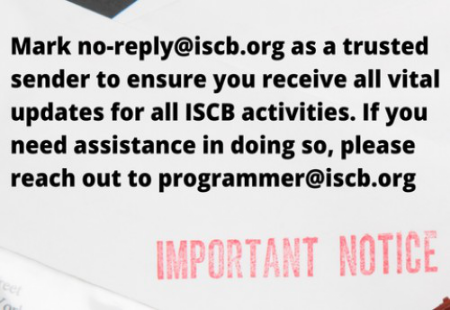The image depicts a photograph of an important notice, resembling a piece of mail or a poster, set against a predominantly white background. In the center of the image, black text reads: "mark no-reply at iscb.org as a trusted sender to ensure you receive all vital updates for all ISCB activities. If you need assistance in doing so, please reach out to programmer at iscb.org." An inverted black triangle appears at the upper left corner, while a red hand-stamped message labeled "IMPORTANT NOTICE" is prominently placed at the bottom right. Additional small details include a white rectangle on the bottom left and a hint of a brown right-angle shape, suggesting the paper might be lying on a desk.